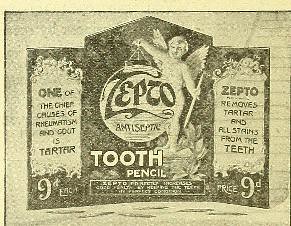This image is a black and white vintage advertisement, likely a newspaper clipping, for the brand Zepto. The central focus of the poster is a winged baby, resembling an angel, holding a circular object with the brand logo "ZEPTO" written on it. Beneath this image, the product name "Tooth Pencil" is displayed in white text. The advertisement appears to be divided into three panels. The left panel reads, "One of the chief causes of rheumatism and gout is tartar." The right panel details the product's benefit, stating, "Zepto removes tartar and all stains from the teeth." The price of the product, listed as 9D, is mentioned at the bottom of both the left and right panels. The background of the image is light grey, adding to the vintage aesthetic of the poster.